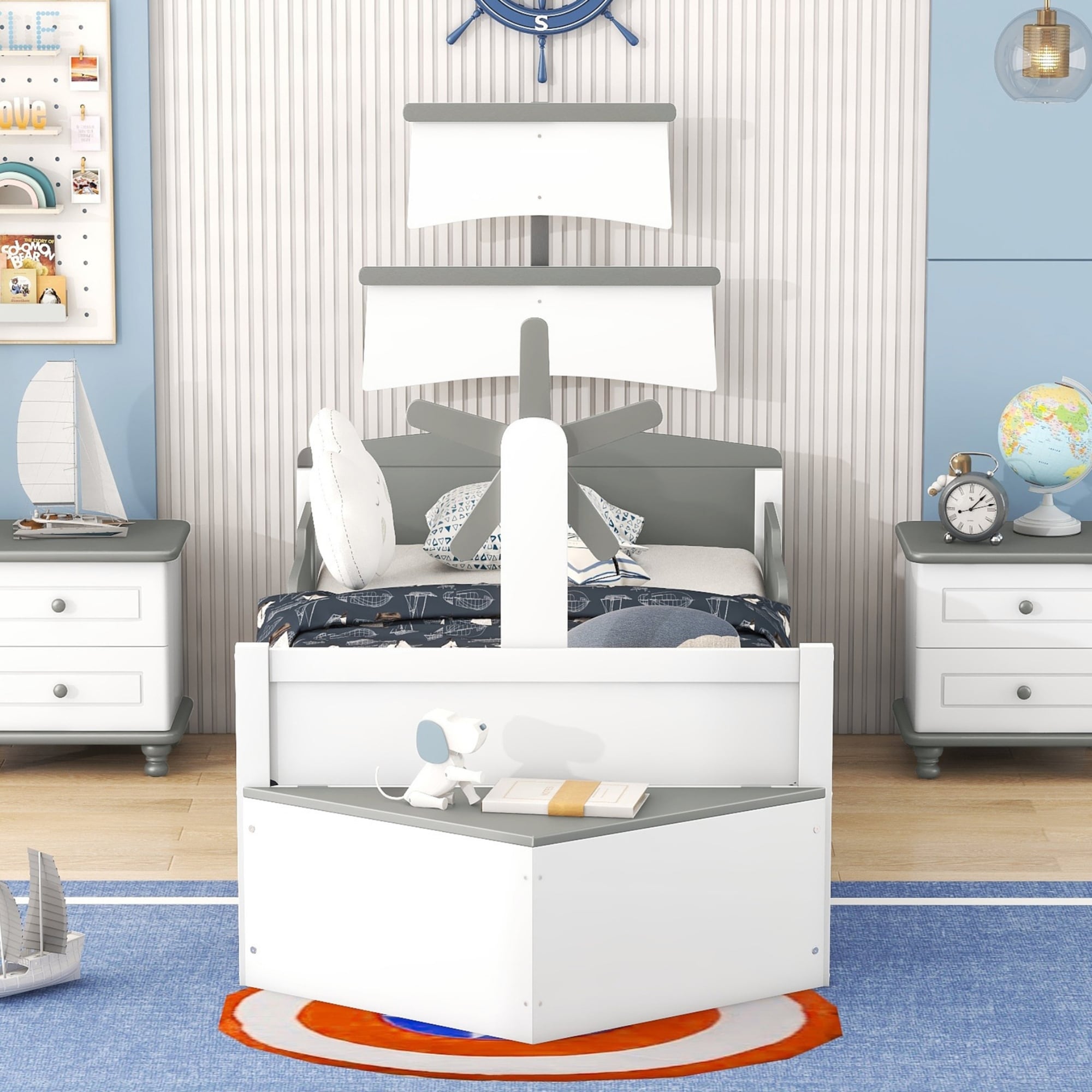This photograph depicts a child's nautical-themed bedroom, centered around a unique bed styled like a sailing ship. The bed is predominantly white with blue and white pillows and a dark blue bedspread adorned with nautical decorations. Above the headboard, there's a mast with two white sails and a boat steering wheel labeled with the directions north, south, east, and west, featuring blue handles.

Flanking the bed are two white nightstands with gray covers and knobs. The left nightstand displays a model sailboat, while the right supports a gray alarm clock and a globe. At the foot of the bed, there is a propeller design, and beneath it lies a blue carpet with a white border and a central red and white target.

The room's background includes walls covered in gray and white with horizontal stripes resembling sails. The floor is a light brown wood, enhancing the nautical ambiance. Additionally, a white bureau engraved with maritime details stands on the left, topped with another model sailboat. A triangle shelf at the foot of the bed holds a white stuffed dog and a white book, completing the room's charming and cohesive theme.